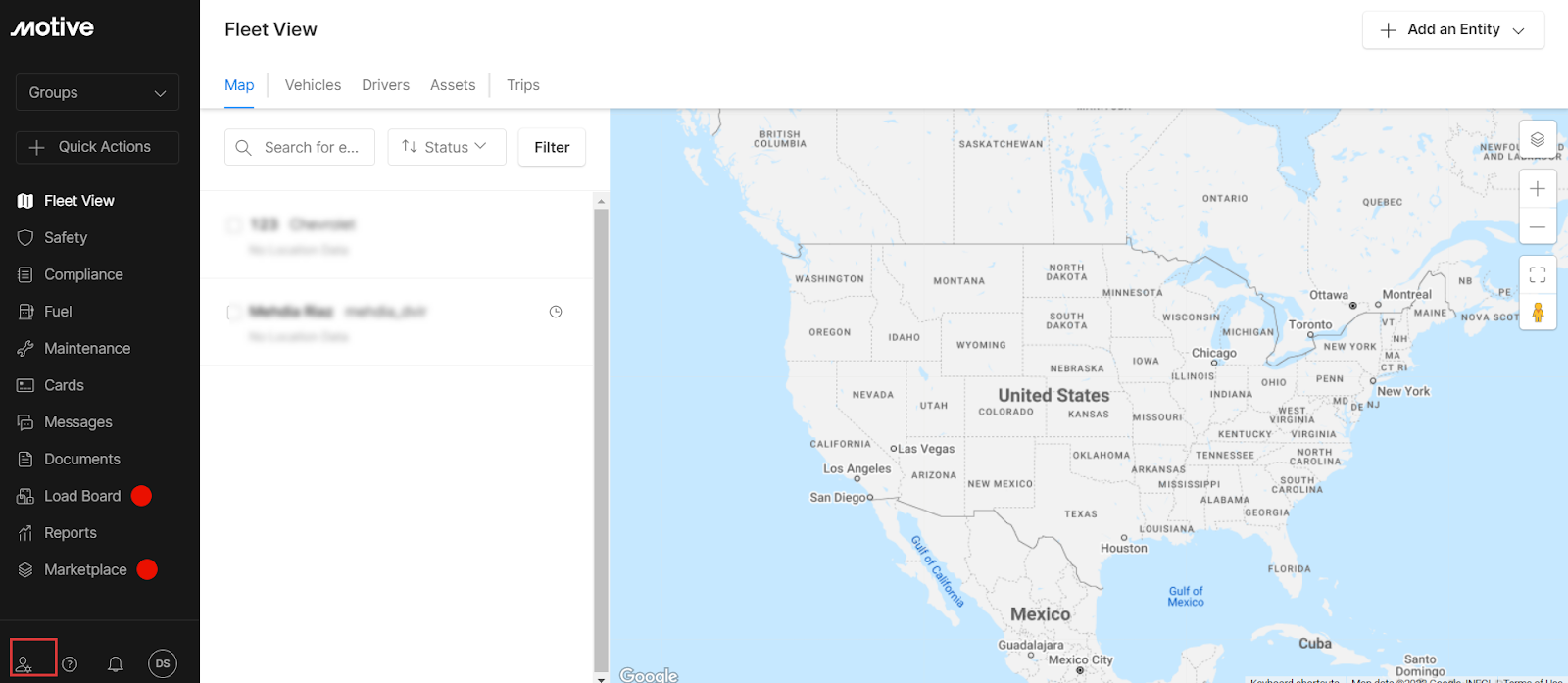In this image, we are presented with a map of the United States, Mexico, and Canada. The map features a blue ocean backdrop and is predominantly white, with state and country names written in black text. 

In the top left corner, the website’s name, "Motive," is prominently displayed in white text. Directly below it, within a boxed area, is the label "Groups." Further down, also in a boxed area, is a plus sign accompanied by the words "Quick Actions." 

A vertical list of categories extends downward from this section, starting with "Fleet View" at the top and followed by "Safety," "Compliance," "Fuel," "Maintenance," "Cards," "Messages," "Documents," "Load Board," "Reports," and "Marketplace." 

At the very bottom left of the image, there are four icons: a person silhouette, a circle with a question mark, a bow icon, and a circle containing a letter.

To the left of the map and extending slightly above it, the heading "Fleet View" is visible. Just beneath "Fleet View," additional categories are listed, including "Categories," "Map," "Vehicles," "Drivers," "Assets," and "Trips."